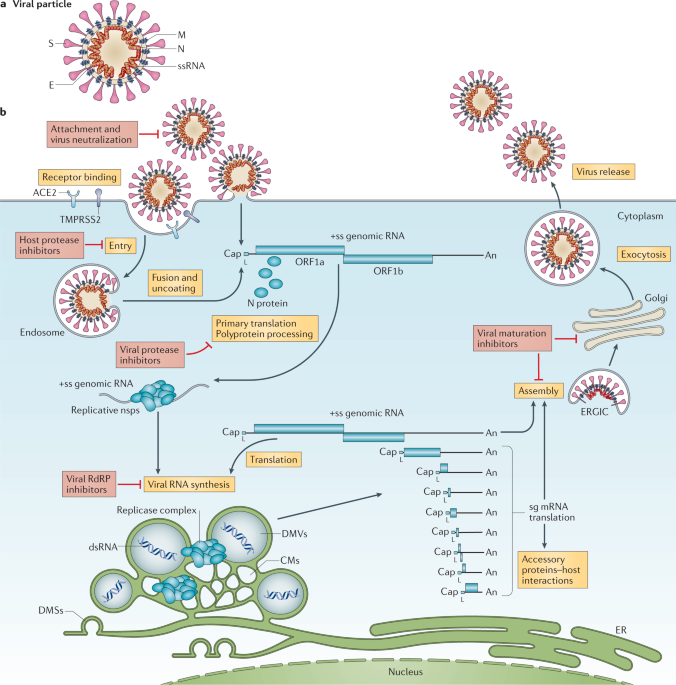The image features a detailed diagram illustrating the life cycle of a virus, specifically depicting the process of viral infection. At the top left, labeled as figure "A," is an illustration of a coronavirus particle, characterized by a roundish brown area housing round pink spores in its outer layer, with an internal structure featuring a blue line and an orange area. Below this, in figure "B," the diagram expands to show the stages of the virus infecting host cells.

A gray horizontal line divides the diagram, with the lower half shaded light blue, representing the host cellular environment. The viral particles are seen entering this blue area through the gray boundary, demonstrating the initial stages of infection. Numerous labels detail the steps and processes occurring, including attachment, virus neutralization, receptor binding, host protease inhibitors, entry, fusion, and uncoating. Additional stages of the viral life cycle are also depicted: primary translation polyprotein processing, viral RDRP inhibitors, viral RNA synthesis, translation, viral maturation, assembly, accessory proteins interactions, host interactions, exocytosis, and ultimately, virus release.

A pale red box to the right of figure "B" emphasizes the processes of attachment and virus neutralization, bordered by a golden rectangle at the bottom. The comprehensive set of labels and visual elements collectively illustrate the mechanisms through which the virus infiltrates the host, replicates, and propagates, providing a thorough overview of viral replication and interaction with the host cell.